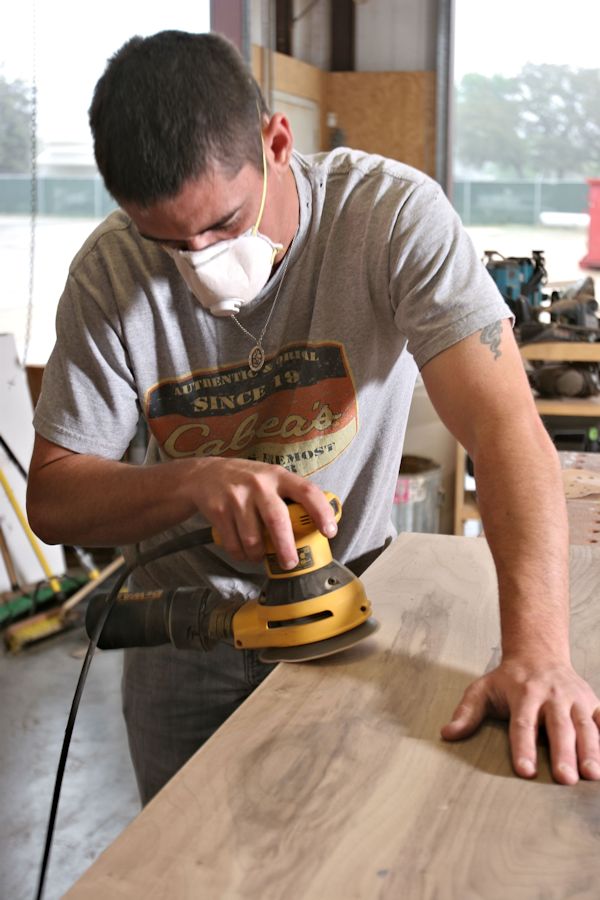In an open, spacious workshop illuminated by natural light streaming through large windows, a focused man in grey jeans and a grey Cabela's t-shirt is captured diligently sanding a flat piece of wood. His short brown hair and a tattoo on his left arm are visible as he leans over his work, bare hands steadying the wood. The man, a white individual, wears a white N95 mask with a yellow strap to protect himself from fine dust particles, and a silver necklace with a medallion featuring a hint of gold around his neck. He uses a small, plug-in rotary sander that is yellow and black. Behind him, an assortment of tools, a red dumpster, a garbage can, and a couple of push brooms are neatly arranged, hinting at a well-organized workspace. The garage door, opened by a chain mechanism, sets the scene for a day of craftsmanship and focus.